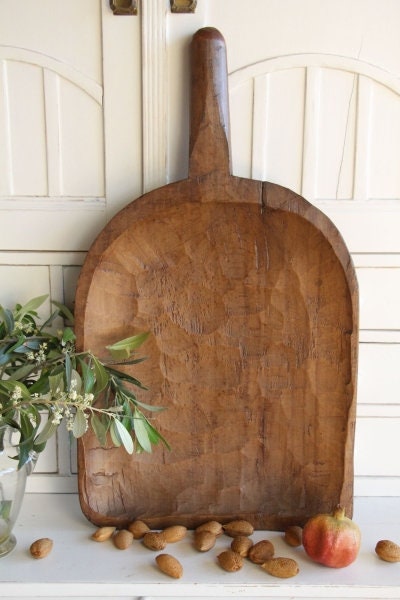This photograph features a rustic, French country style wall composed of small white wooden planks with two brass knobs. Leaning against the wall is a roughly hand-carved, u-shaped wooden board with a handle at the top, resembling a large paddle or pizza tray. The wooden piece displays an uneven, scooped-out surface, highlighting its artisanal craftsmanship. In front of the board, scattered across the countertop, are an assortment of brown nuts, likely almonds, and a slightly shriveled, red pomegranate. To the left, partially visible, is a glass vase containing greenery with muted, grayish-green to dark green leaves, adding a touch of natural decor. The entire scene is set against a white backdrop, suggesting it is propped up against some cupboards.